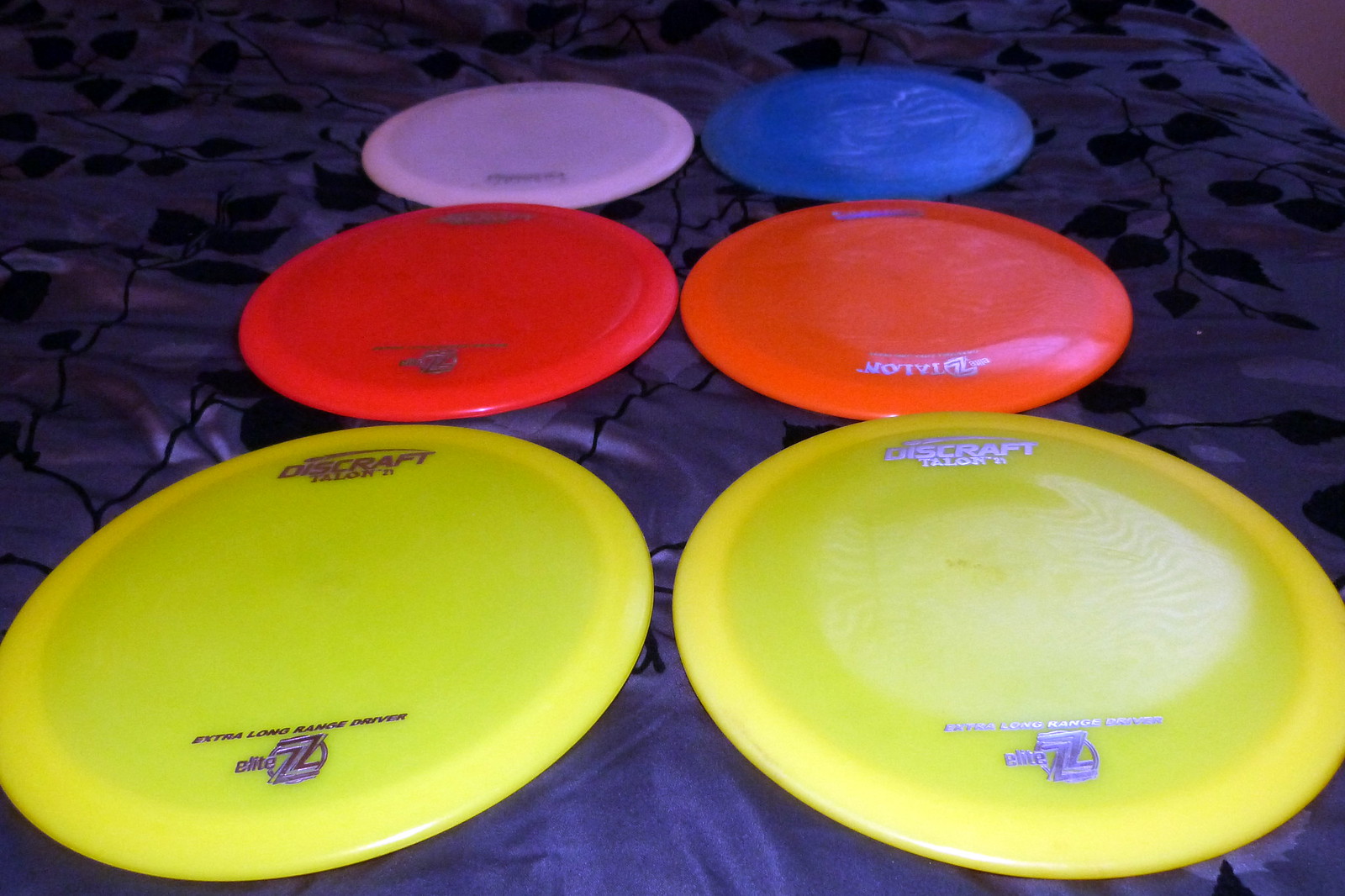This color photograph features six Discraft frisbees meticulously arranged on a surface that appears to be a bedspread. The bedspread is made from a silky, purple material adorned with black vine and leaf patterns. The frisbees are organized in three rows of two. Starting with the top row, the frisbee on the left is light purple while the one on the right is blue. The middle row features a red frisbee on the left and an orange one on the right. The front row displays two yellow frisbees. Each frisbee boasts the Discraft logo, with additional writing near the top that is too blurry to be clearly legible. The frisbees in the foreground look larger due to the close-up perspective of the photo.